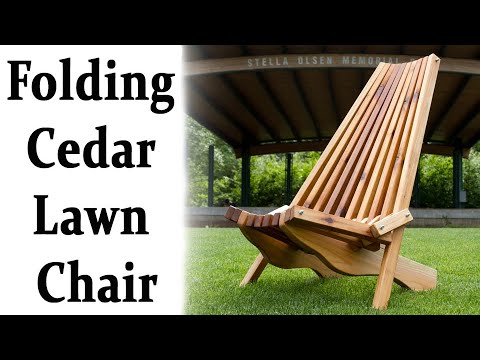The photograph showcases an advertisement for a folding cedar lawn chair set against a beautifully manicured green lawn. The chair, intricately crafted from cedar wood, features a unique design with a notably long backrest composed of vertical slats that widen towards the seat and narrow near the top, forming an almost triangular shape. The chair's design allows for a reclined lounging position, ideal for comfortable outdoor relaxation. The backdrop shows a pavilion, labeled the "Stella Olson Memorial," providing a protected area with a roof structure. The pavilion is surrounded by lush, full trees, further enhancing the serene outdoor setting. The text "Folding Cedar Lawn Chair" is prominently displayed on the left side of the advertisement in a white background with black lettering. The overall scene suggests a tranquil, inviting environment perfect for enjoying the outdoors.